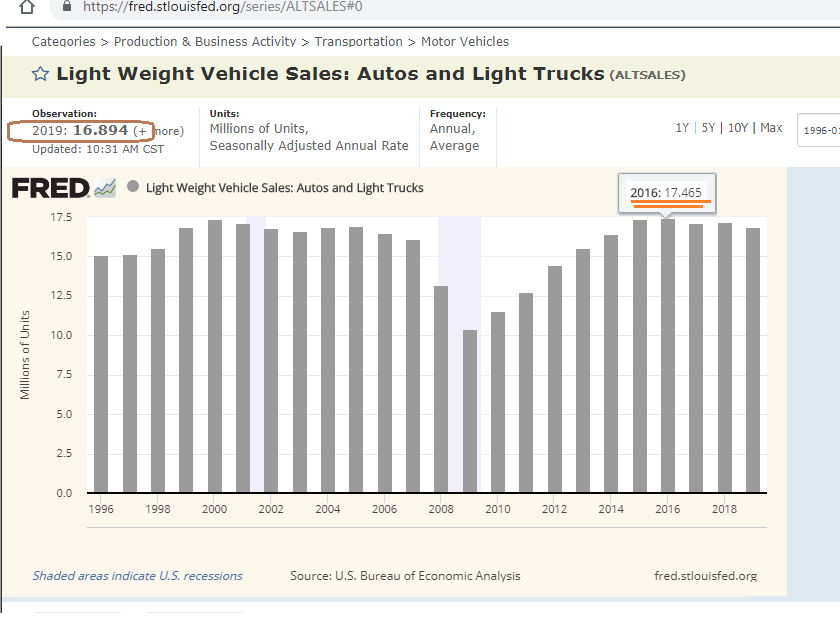The image is a screenshot of a graph from the website fred.stlewisfed.org, detailing "Lightweight Vehicle Sales, Autos and Light Trucks" from 1996 to 2018. The vertical axis ranges from 0 to 17.5 million units, representing the seasonally adjusted annual rate of vehicle sales. Key data points are highlighted: an average of 17.465 million units sold in 2016 and 16.894 million units in 2019. The graph, sourced from the U.S. Bureau of Economic Analysis, also shows a notable decline in sales during 2008, 2009, and 2010. The data is presented in a bar graph format, with the latest update recorded at 10:31 AM Central Standard Time.